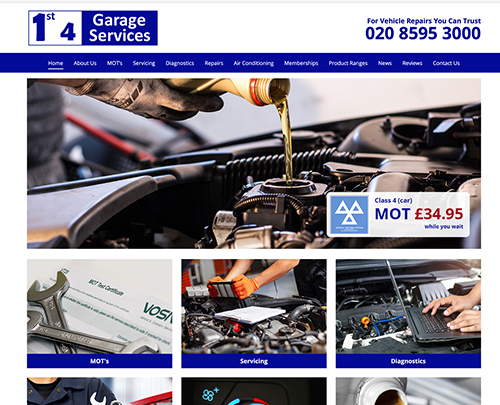The image displays the homepage of a website for a garage service company. At the top right corner, there is a blue logo accompanied by a phone number. The homepage features a navigation bar with multiple options, set against a blue background. Several images are prominently shown: mechanics working on cars, one pouring oil into an engine. There is a promotion in red text, though it is slightly unclear, it appears to state "$34.95." This promotion is prominently placed towards the front.